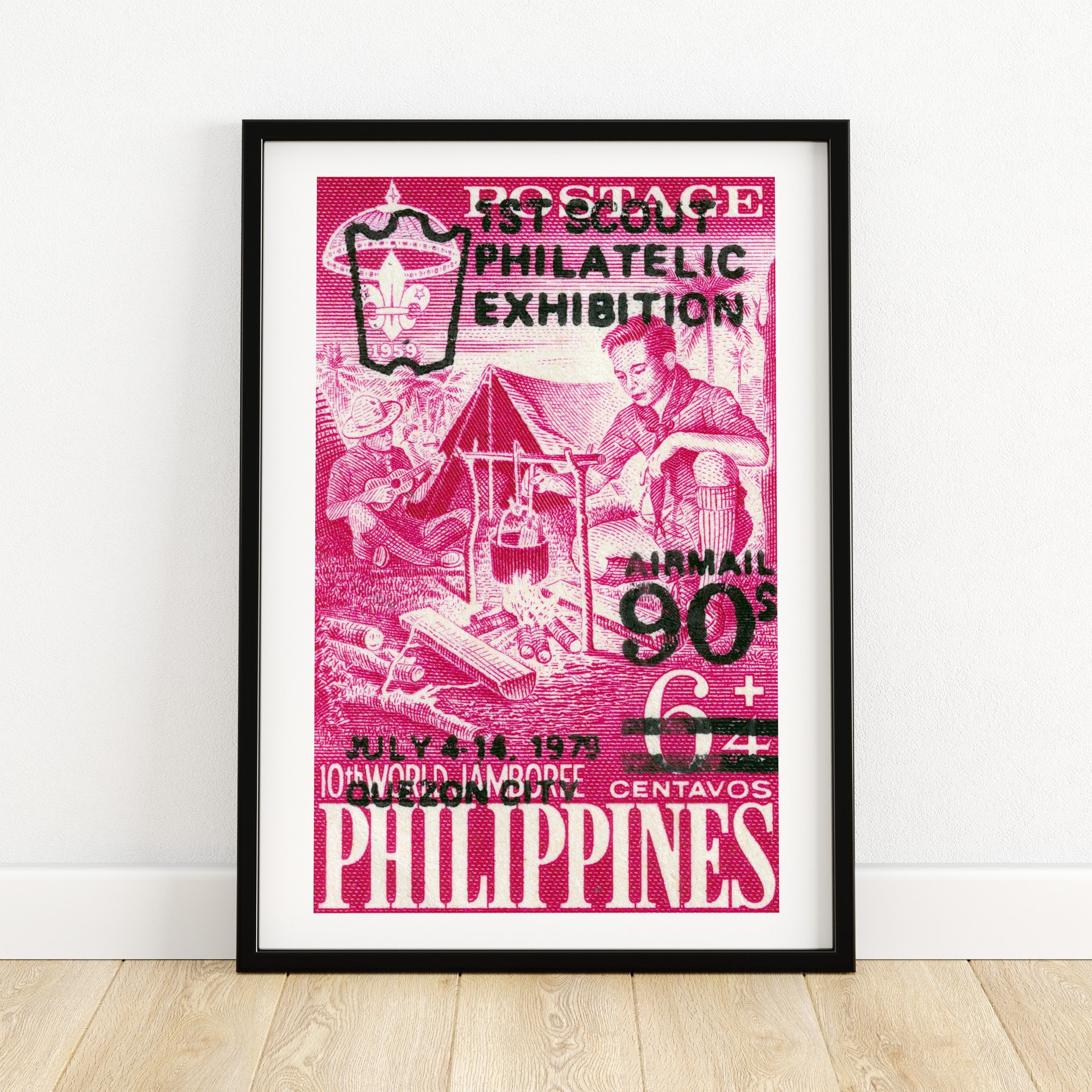This photograph showcases a framed, enlarged image of a postage stamp, set against a pale hardwood floor with white baseboards and a white wall. The black rectangular frame rests on the floor, leaning against the wall. Inside the frame is a white mat, encasing the enlarged stamp, predominantly featuring a reddish-pink hue with highlights of white. The stamp depicts an illustration of two men in uniforms at a campsite. On the right, a man kneels, holding a spatula and interacting with a black pot suspended over a campfire. On the left, another man, donning a round, white ranger hat, plays a small ukulele. A pup tent can be seen in the background.

The stamp includes various inscriptions: "postage" in white text at the top, accompanied by a fleur-de-lis and the year "1959." Overlaying the stamp in black text, it reads "First Scout Philatelic Exhibition," followed by "Air Mail 90S" and the date "July 4, 14, 1979, Quezon City," flanked by two black horizontal lines. White text at the bottom left states "10th World Jamboree," with "Philippines" prominently displayed below. Additionally, "6 plus 4 centavos" is noted on the right side over "Philippines."